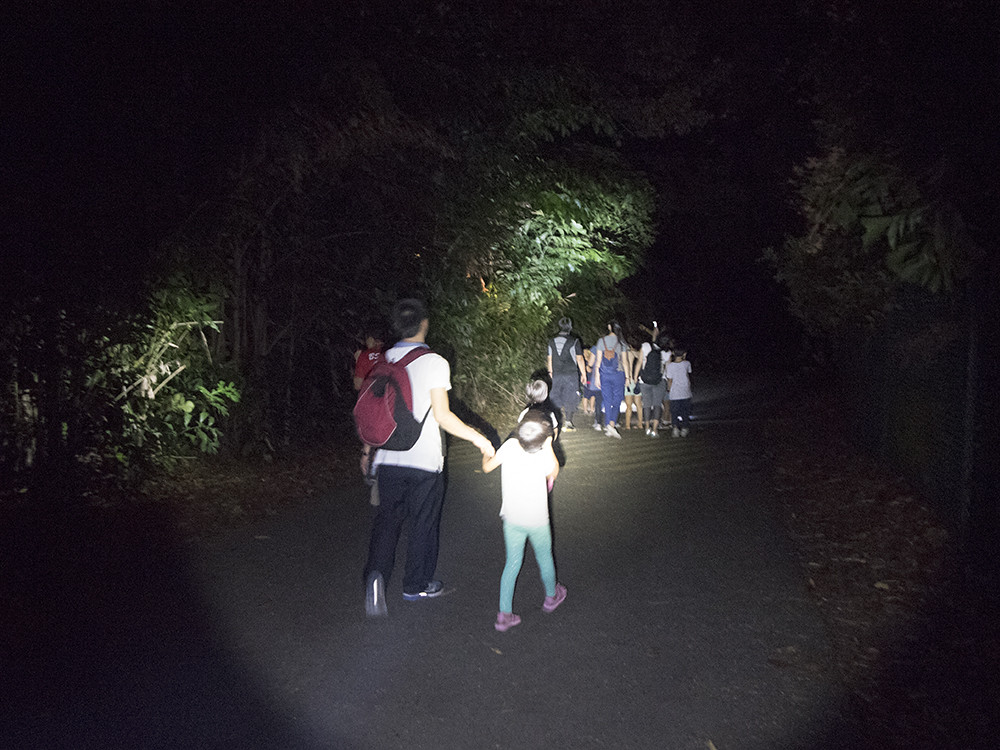In the photograph taken at night, a man dressed in a short-sleeved white shirt, black pants, and carrying a maroon and black backpack is seen on the left side of a dark asphalt path, holding the hand of a young girl wearing a white t-shirt, teal-colored leggings, and pink shoes. The entire group, composed of several adults and children, are walking away from the camera, with their backs to the viewer. The path, likely made of asphalt, is surrounded by thick trees and shrubs on both sides. The scene is illuminated by a flashlight, creating a circular area of light in the center of the image while the edges remain shrouded in darkness. In the distance, another larger group of three adults and several children can be seen further down the path. The entire area within the flashlight's beam is revealed in clear contrast to the dark surroundings, highlighting the trees and the group ahead.